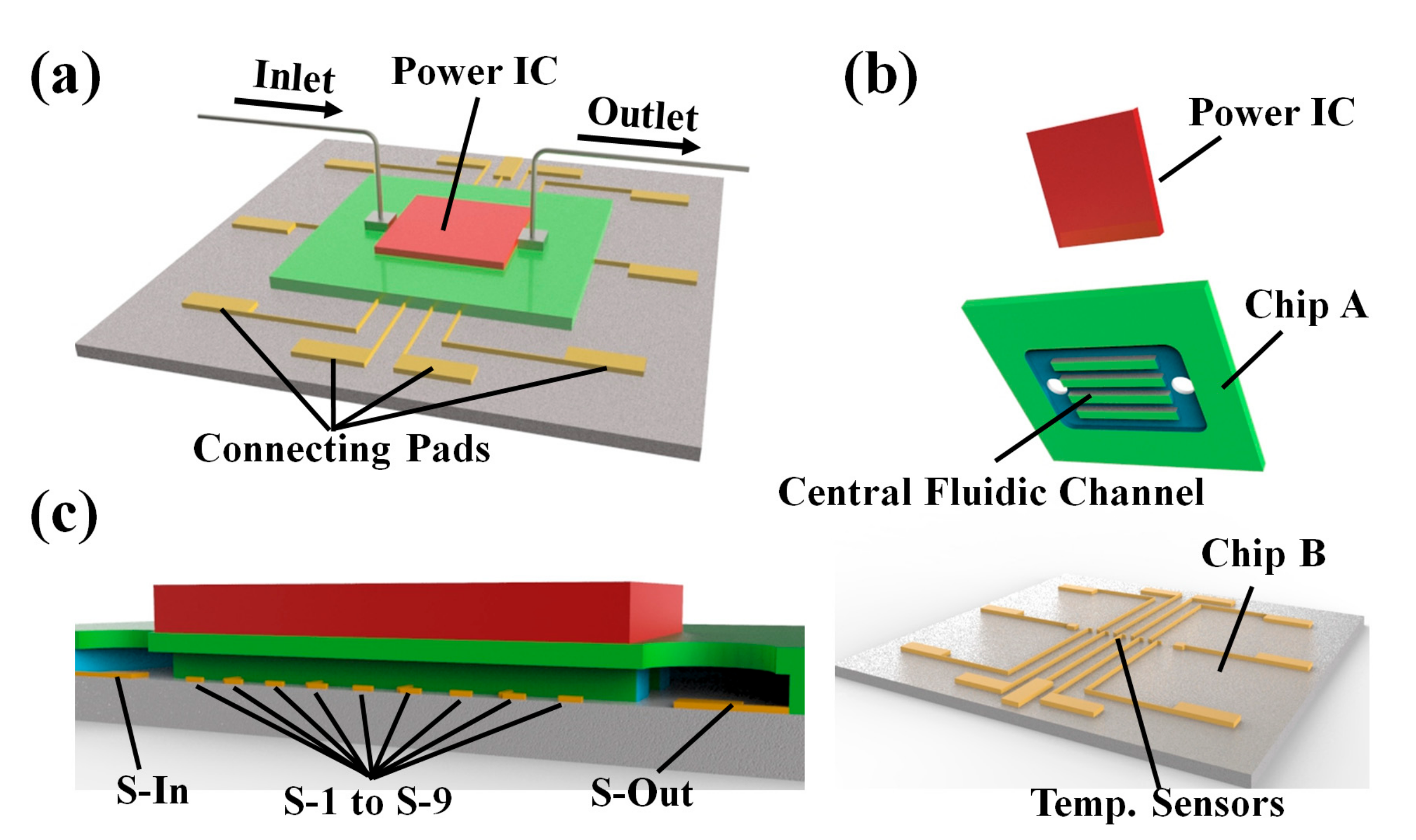This image is a detailed diagram, featuring four parts arranged in a 2x2 grid against a white background, with the bottom right one unlabeled. The top left section is labeled A, showcasing a black or gray square with yellow connecting pads, a green square, and a smaller red square labeled Power IC. It includes labeled components such as Inlet, Outlet, and Connecting Pads made from gold. The upper right section, labeled B, depicts a green board labeled Chip A, with a red Power IC atop it, showing its internal structure including a central fluidic channel. The bottom left section, labeled C, provides a side view of the whole assembly, illustrating the biome with labels like S In, S1 to S9, and S Out, along with temperature sensors. The components and connections are color-coded for clarity, with gold for connecting pads, silver for inlets and outlets, and red for the Power IC, all laid over a green circuit board. The diagram offers a comprehensive look at the intricate details of the parts and their interconnections.